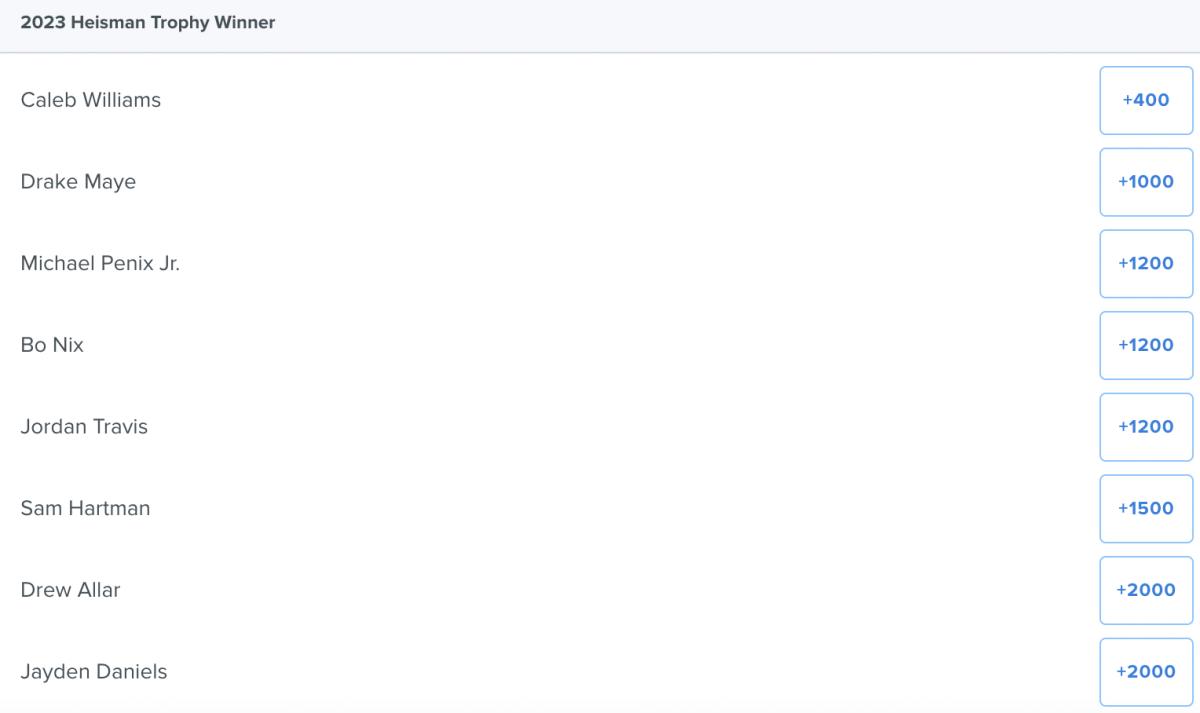This image is a screenshot featuring a list of candidates for the 2023 Heisman Trophy. At the top, the screen displays the title "2023 Heisman Trophy Winner" in black letters. This text is not very large, suggesting that it serves as a header rather than the main focus. Below the title, there is a neatly organized list of eight names, each accompanied by a blue button. Each button has a white background with a blue border, containing a number that indicates the odds associated with the respective candidate.

Here are the listed names along with their associated odds:
1. Caleb Williams: +400
2. Drake Maye: +1,000
3. Michael Penix Jr.: +1,200
4. Bo Nix: +1,200
5. Jordan Travis: +1,200
6. Sam Hartman: +1,500
7. Drew Allar: +2,000
8. Jayden Daniels: +2,000

The presence of the odds next to each name suggests that this screenshot might be from a betting site or a platform that provides predictive analytics for the Heisman Trophy winner, although the image itself does not specify this.